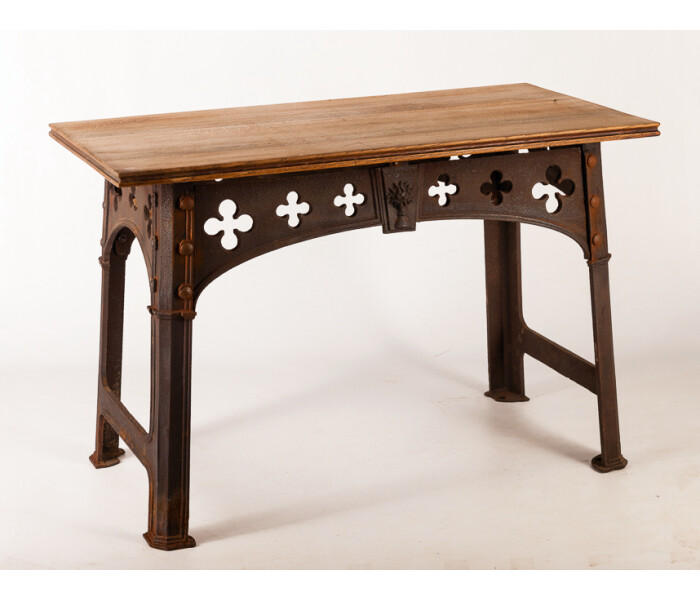This photograph showcases an antique table set against a stark white floor and background, giving it a striking contrast. The table features a rectangular wooden top that appears relatively newer compared to the rest of the structure. Supporting the top are four cast iron legs that show signs of slight rust, emphasizing the piece's age. While the legs themselves are not highly intricate, there are decorative cutouts resembling plus signs or old crosses—six along each longer side and three at each end. These cutout designs add a unique, vintage charm to the table. The table's bolts, which securely attach the wooden top to the iron legs, are large and circular with notable rust, further highlighting its antiquity. The overall appearance of the table suggests it could be a treasured piece from a bygone era, with both rustic and historical appeal.